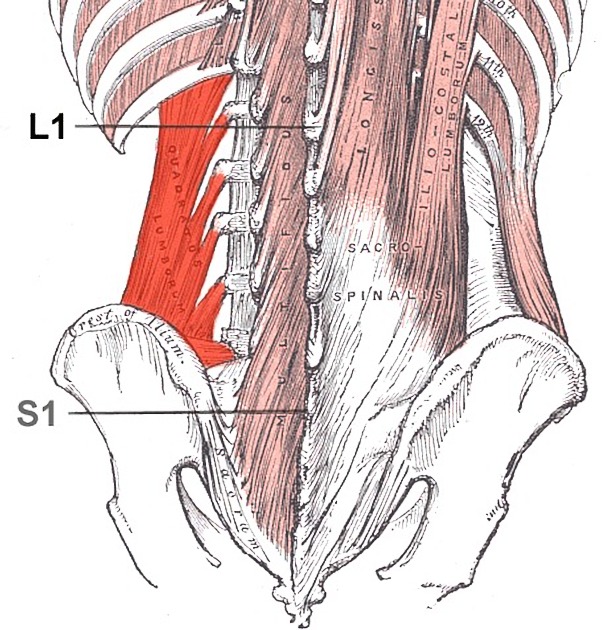This detailed infographic is an old-fashioned medical drawing, sketched in black and white, depicting the lower spine, hip bones, and respective muscles. The illustration spans from the pelvis up to the middle of the ribcage, featuring both skeletal and muscular structures. The musculature is highlighted in shades of pink to red, indicating varying depths of connective tissue, with deeper structures in dark red. Key anatomical parts are meticulously labeled: the 10th, 11th, and 12th ribs are marked out horizontally; L1 and S1 are indicated with black directional lines. Annotations also include "sacro," "spinalis," "iliocostal," and "lumborum," clearly identifying specific muscle regions and ligaments. The ribcage and pelvis are distinctly shown, providing a comprehensive view of the lumbrosacral area.